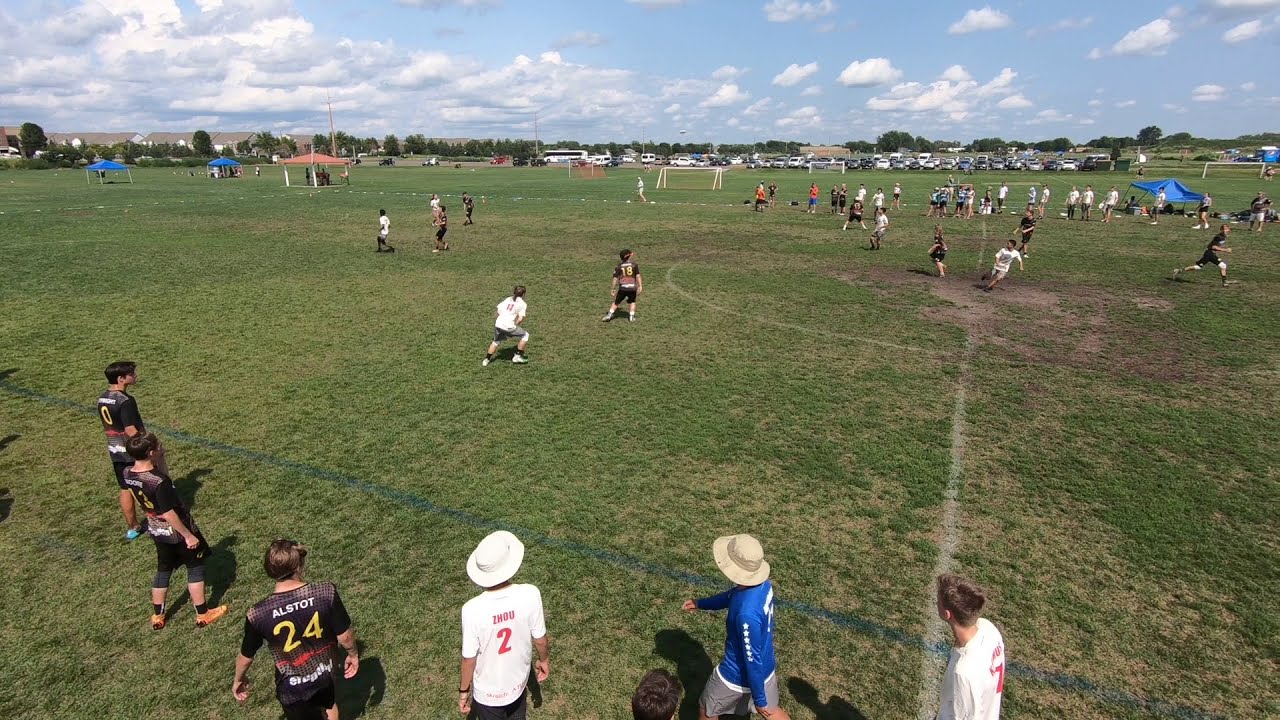Captured during a partly cloudy daytime, this photograph showcases an outdoor soccer event on a large, grassy field meticulously sectioned with chalk lines. The scene is bustling with activity: numerous players dressed in two distinct uniforms—white and black—are spread across the field, actively participating in the game. Along the bottom of the image, some players in black uniforms with green numbers sit or stand, awaiting their turn, while spectators are gathered just beyond the sidelines. The field is set against a backdrop of blue tents and peach-colored tents with roofs, all under a sky dotted with white and gray clouds. A line of trees demarcates the horizon, behind which a parking lot filled with cars is visible, reflecting the significant turnout for the event.